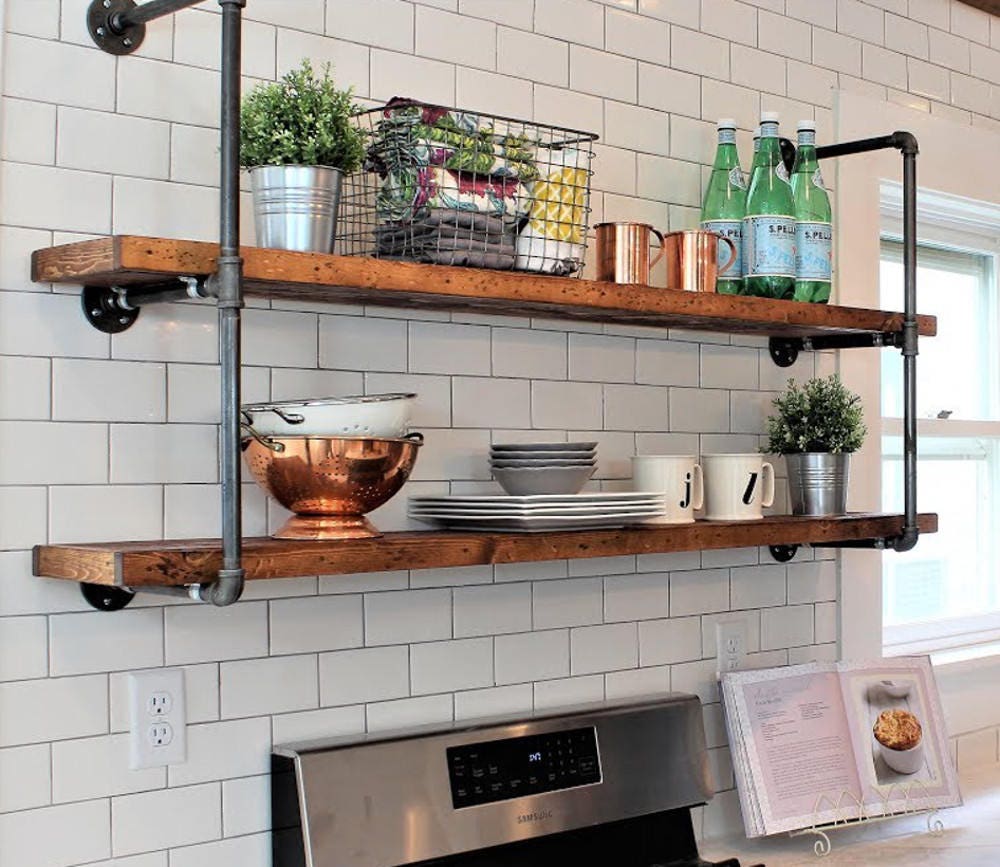This photograph captures an organized and well-styled kitchen scene featuring two wooden shelves mounted on a white, smooth brick-patterned wall, supported by black metal stanchions. The shelves hold a variety of carefully arranged items, including a silver pot with green plants, folded wooden slats in a basket, bottles of sparkling water, colanders in white and gold, plates, mugs, cups, containers, and a crate. At the bottom of the image is a grey and black stove with a digital clock displaying 1:47, adjacent to an open recipe book. To the right side of the image, a closed window with white trim allows bright light to filter into the cozy, inviting space.